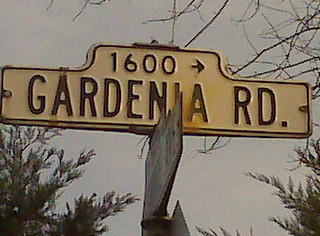In this low-resolution photograph taken on a dim day, the scene features partially leafless green trees framing the edges. At the center stands an aged metal street sign. The sign is yellow with faded black or dark brown lettering. It reads "Gardinia Road" and includes the number 1600, with an arrow pointing to the right. The nostalgic feel of the sign adds a touch of vintage charm to the otherwise dull and overcast environment.